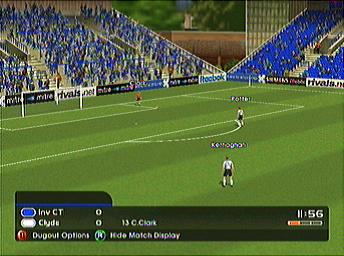A nostalgic screenshot from a vintage video game captures a classic soccer match on a lush green pitch. The screen shows a section of the field with the white penalty box clearly outlined. Three players are visible: two wearing white jerseys paired with black shorts, and one in a red uniform. Though the players' names appear above them in white text, they are not legible. Below the action, a rectangular heads-up display shows team names and the game timer (11:56) against a black background. The bleachers in the top left and right are filled with a largely blue crowd, while the net of the goal is faintly visible in the top left corner. The graphics, reminiscent of the early PlayStation era, are grainy and lack modern detail, giving the scene an endearing, retro charm. Vibrant splashes of blue and white are visible at the bottom left, contrasting with a hint of orange on the bottom right.